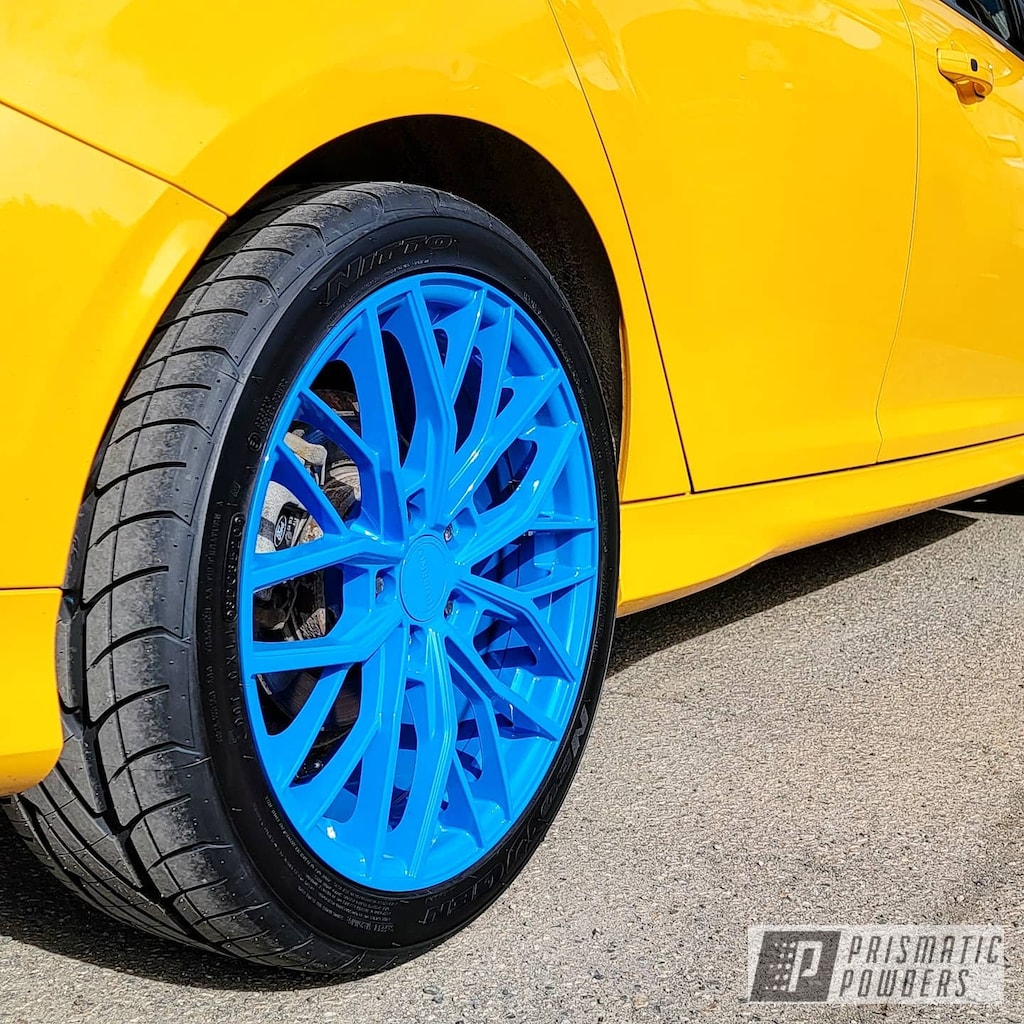The image captures a close-up of a bright lemon-yellow car, focusing primarily on the lower rear passenger side and its wheel. The wheel, which features a black tire with visible tread wear, is adorned with a bright blue rim showcasing a geometric interlocking design. The car's shiny, new exterior emits a reflective sheen, indicating on a bright, sunny day. The vehicle is parked on a pavement, casting a distinct shadow. In the lower right corner of the image, a watermark displays the text "Prismatic Powers" alongside a stylized 'P' emblem, suggesting the image might be an ad for a tire company. The vehicle’s sporty, low-to-the-ground design hints at its high-performance nature.